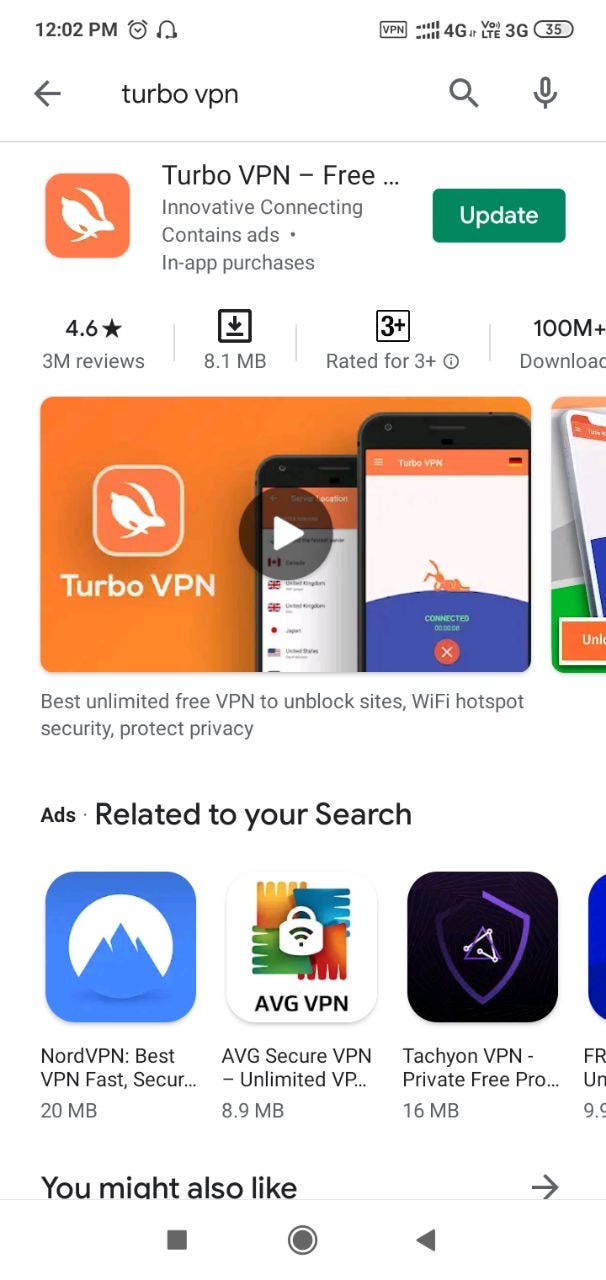The image depicts a screenshot taken from a smartphone, displayed against a plain white background. In the upper left corner of the screen, the time is shown as 12:02 p.m. Adjacent to the time, there is a series of icons: an alarm clock, a pair of headphones, and a VPN symbol. Further right, signal strength bars are visible, indicating 4G connectivity. The acronym "VOLTE" appears stacked vertically, and beside it, "3G" is shown. Finally, the battery icon displays a 35% charge.

Moving below, on the left side, there's a black left-pointing arrow and the text "TurboVPN." On the far right of this section, there's a search icon (magnifying glass) followed by a microphone icon, separated by a gray dividing line.

The main content of the screen shows a selected application, "TurboVPN Free," which is represented by an orange square icon featuring a white rabbit. The app's description states "Innovative connecting, contains ads, in-app purchases." A green "Update" button is positioned to the right. Additional details indicate a rating of 4.6 stars from 3 million reviews, a download size of 8.1 megabytes, an age rating of "3+," and over 100 million downloads. A video thumbnail below this information features the TurboVPN logo and two smartphones, with the tagline "Best Unlimited Free VPN to Unblock Sites, Wi-Fi Hotspot Security, Protect Privacy."

Below the main section, there's a heading labeled "Ads related to your search," showcasing three apps. The first is NordVPN, identified by a blue mountain and white moon logo on a blue icon, described as "Best VPN, Fast Security," with a size of 20 megabytes. The second app is AVG Secure VPN, displaying a plaid background with a white lock and Wi-Fi bars, labeled "AVG VPN" and sized at 8.9 megabytes. The third app is Tachyon VPN, identified by a black icon with a purple shield outline and white triangle logo, described as "Tachyon VPN Private Free Pro," sized at 16 megabytes.

Finally, at the bottom, there's a section titled "You might also like," with an arrow pointing right, followed by the standard mobile navigation icons: a square, a circle, and a triangle.